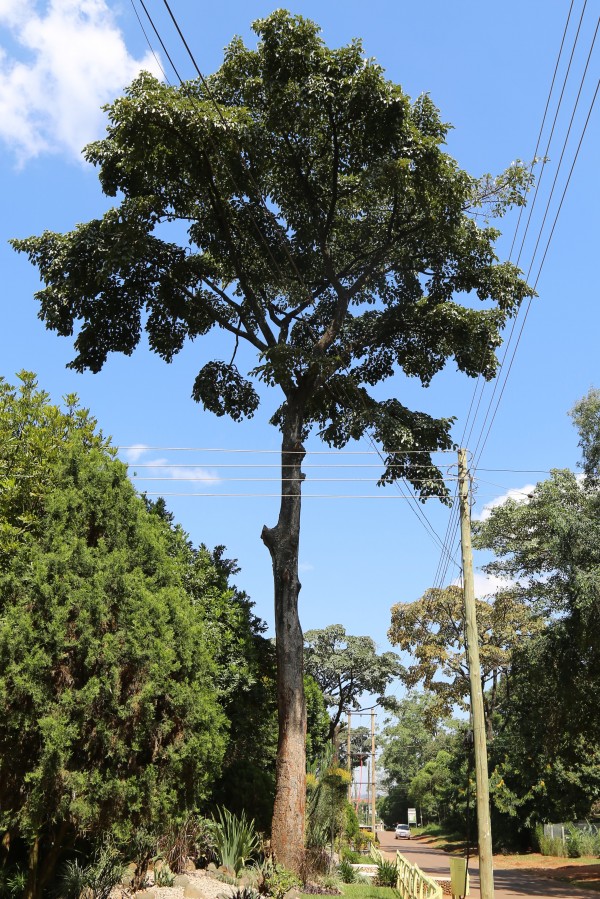This is a color portrait-layout photograph focusing on an exceptionally tall tree with a slender trunk and a lush, circular canopy of green leaves. This towering tree notably surpasses the height of the surrounding telephone poles and power lines, which crisscross the image. The sky in the upper background is a vibrant blue adorned with scattered white clouds. In the bottom left, dense foliage, bushes, and grass open up the scene. The bottom right reveals a street with a distant white car, flanked by more greenery and a chain link fence. No people or text are visible, emphasizing the solitary grandeur of the tree within this suburban environment.